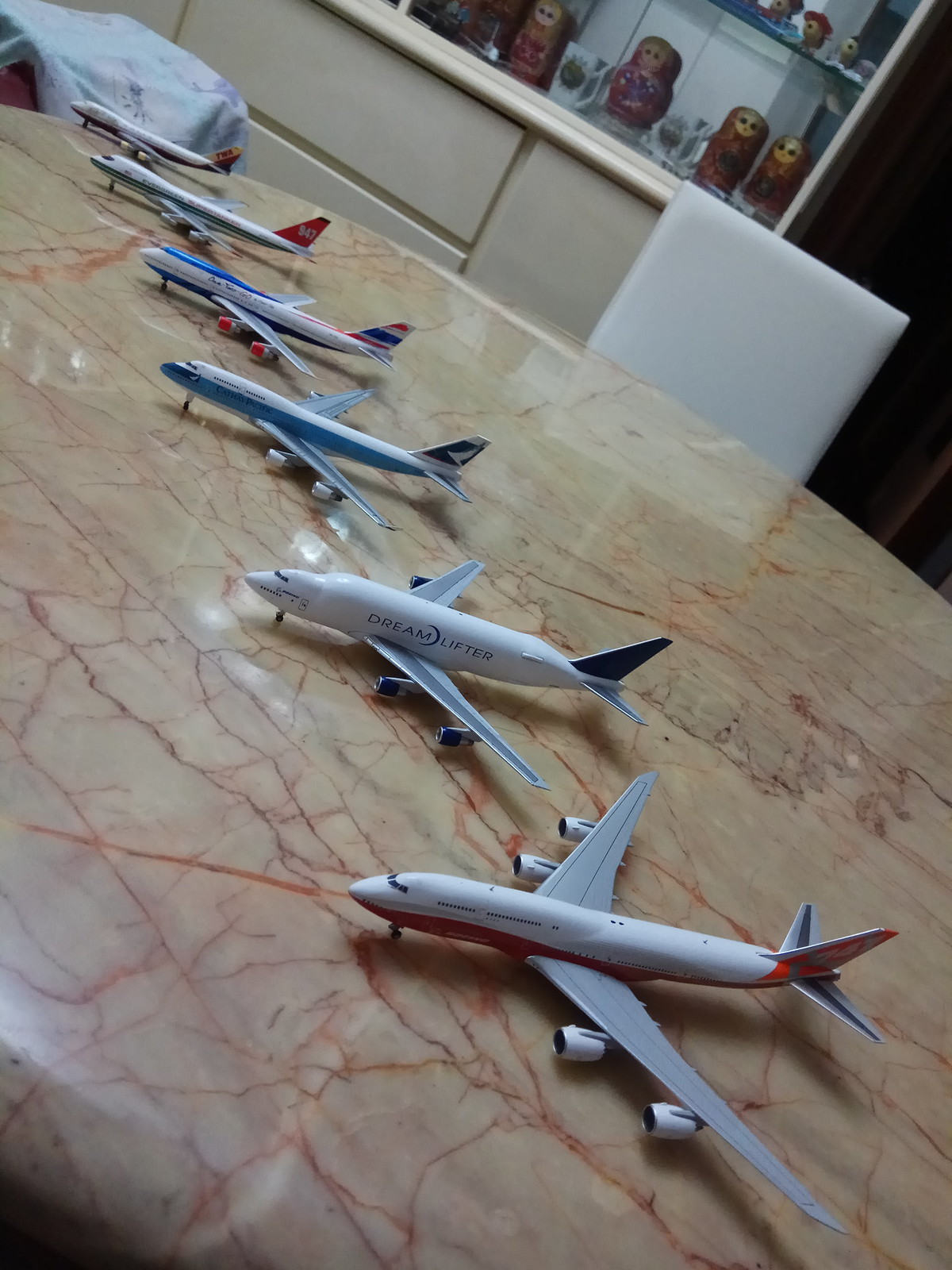The image portrays a collection of six model jetliner airplanes aligned in a single row atop a cream-colored marble table, streaked with intricate veins of reddish-orange, brown, and hints of green. Captured from a diagonal perspective, the scene extends from the bottom right to the top left, with the larger planes positioned closer to the viewer and progressively smaller ones towards the back. The predominantly white airplanes feature blue and red accents, creating a uniform aesthetic. In the background, the upper part of a white chair and a white cabinet with a glass top housing several dolls, including Russian nesting dolls, are visible, adding a touch of domestic charm and nostalgia to the setting.